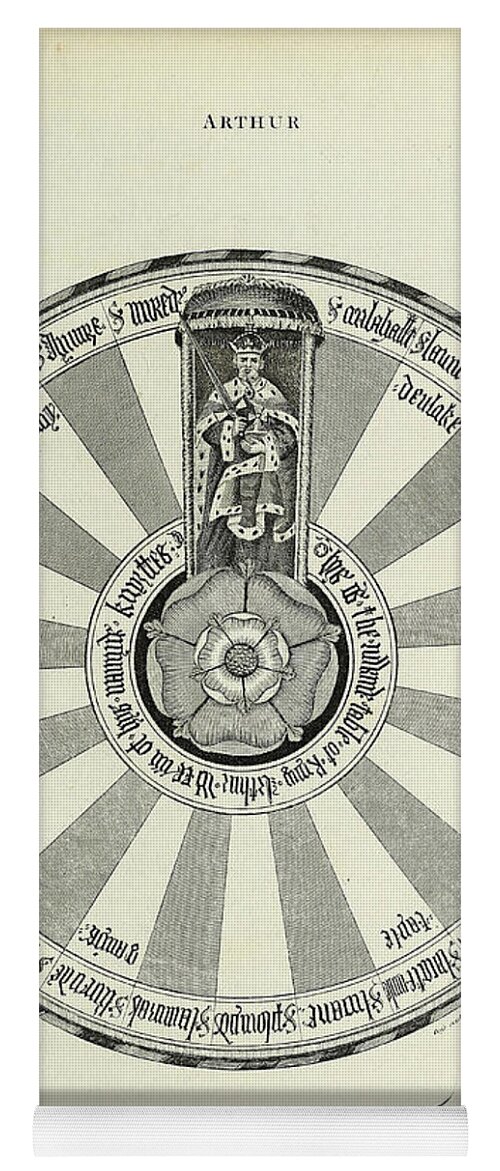This detailed image, reminiscent of an illuminated manuscript from the Medieval Times, prominently features the word "Arthur" in an old-fashioned font at the top. Below this title, the central focus of the image is a large, circular design resembling a dartboard, divided into alternating white and dark gray sections. In the very heart of this circle, there lies a five-pointed flower encircled by an inscription in a fancy, difficult-to-read font, likely in Latin. Above this central flower, within the circle, stands a regal figure — a king, adorned in a crown and royal, fur-covered robes, holding a sword. He is positioned inside a narrow structure that appears to be a throne. His gaze is directed downwards towards the circle’s center. The entire design is monochromatic, consisting of black, gray, and cream hues. Latin words also embellish the outer rim of the circle, further enhancing the medieval aesthetic of this intricate image, which is cut off at the sides, giving the viewer a close-up look at the fascinating details. The segmented sections and inscribed names around the circle likely represent Arthur and his Knights of the Round Table.